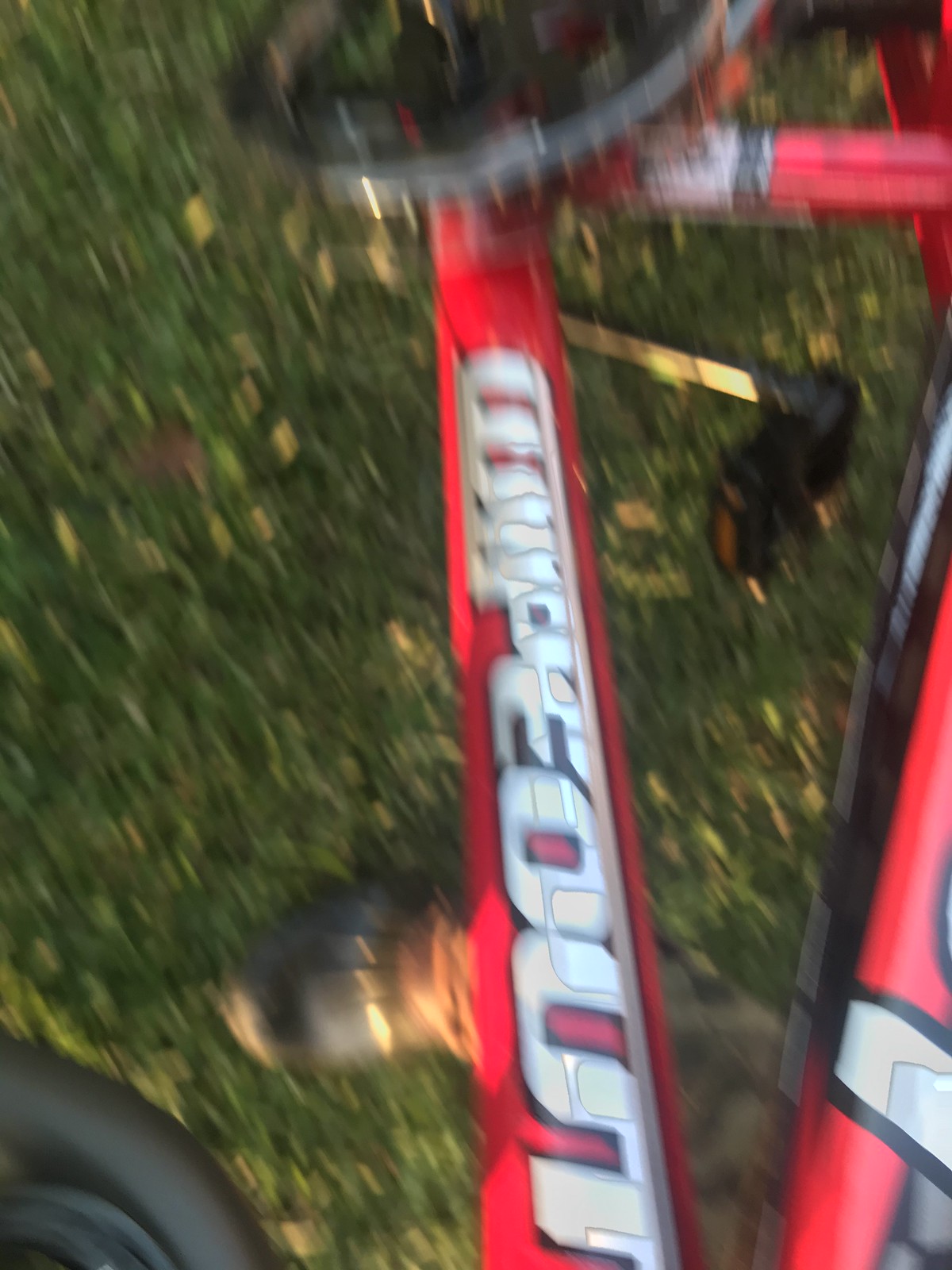The photograph is an extremely out-of-focus image depicting a bicycle laying on the ground. The lower bar of the bicycle frame is somewhat discernible and features text that appears to read "Camp Out," though clarity is compromised. The composition includes part of the bike's gears at the top and the left pedal. The right-hand side shows a portion of a tire, whereas the bottom left corner reveals another tire fragment. Adding to the scene, a person's foot clad in a brown shoe with camo pants and a hard, plastic black front is visible in the lower part of the photograph. Despite the blur, these elements form the composition of the image.